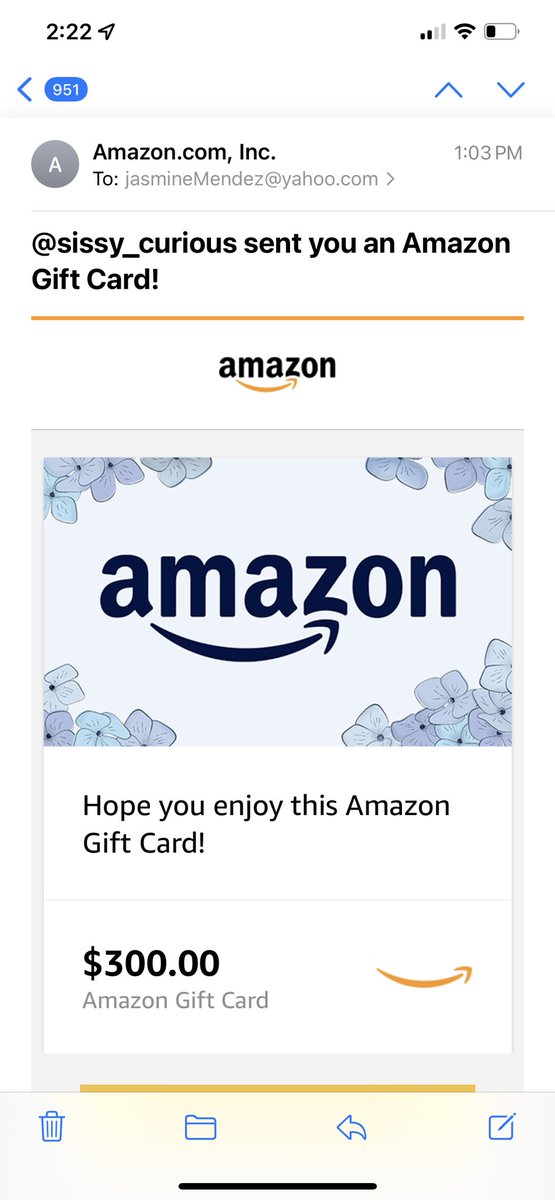This image is a screenshot of an email displaying an Amazon gift card. The photo is in portrait orientation, mimicking the dimensions of a smartphone screen, and lacks defined outside borders. It is primarily set against a white background.

At the top of the screenshot, a thin gray bar acts as a header, displaying essential status indicators. On the top left, the time "2:22" is shown next to an upward-facing navigation arrow. The network status bar indicates a 2 out of 4 signal strength, followed by a fully connected Wi-Fi symbol. The battery icon indicates approximately 25% remaining. To the right of these icons, there is a blue backward caret with a white bubble inside that shows the number "951" in white, flanked by an up-and-down caret symbol.

Below this header, the email displays a gray circle avatar with a white "A" in the center, indicating the sender as Amazon.com, Inc. The recipient is identified as Jasmine Mendez, with the email sent to Jasmine’s Yahoo address at 1:03 PM. The email subject reads, "At Sissy Curious sent you an Amazon gift card."

The main content of the email features a prominent orange horizontal bar with the Amazon logo, followed by a greeting: "Hope you enjoy this Amazon gift card." Below this message is the gift card amount, a generous $300, which stands out. At the bottom right of the email, the Amazon Prime logo is displayed, characterized by a yellow looping arrow pointing to the right.